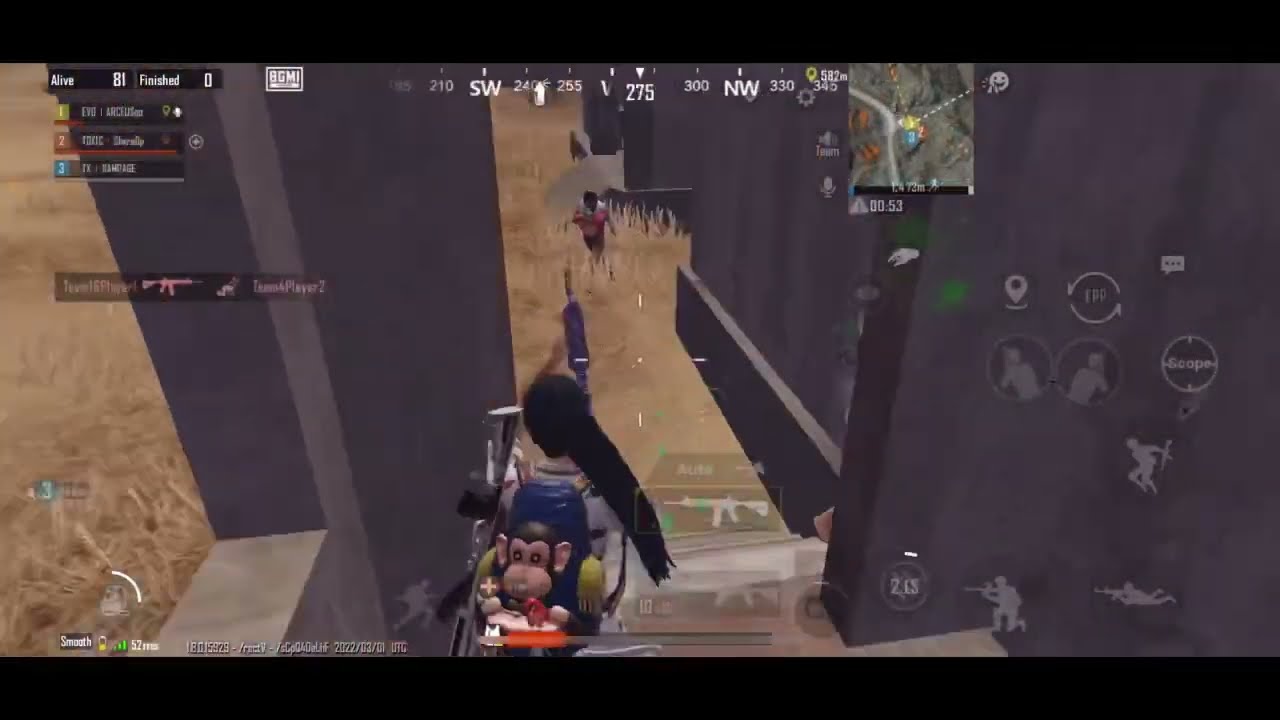This horizontal rectangular screenshot from a video game features a solid black border at the top and bottom, enclosing a scene dominated by gray and brown tones. The setting is a dark gray stone structure that spans both the right and left sides of the image. This stone architecture includes a prominent stairway situated towards the right, with characters placed strategically across it. On the left edge of the scene, brown, straw-like grass is visible, contrasting with the stone.

In the space between the stone structures, a notable character stands out—a monkey facing towards the viewer, adorned with a blue backpack or jacket that has gold officer-like stripes on the shoulders. This character appears to be positioned at the bottom middle of the image. A woman with long, black hair is seen sitting on the stairs, her back to the viewer. Lower down the stairs, another figure can be seen among the grassy area, seemingly approaching the other characters, although details about this figure remain indistinct.

The upper part of the image is laden with numerous elements: a series of numbers and directional labels such as Southwest (SW) and Northwest (NW) span the top of the screen. In the upper left corner, text elements like "Alive 81" and "Finished 0" are partially visible, though some details are blurred. Additional UI elements, such as control panels and possibly a navigational box, are faintly displayed on the right side from the middle downwards, featuring multiple circular icons.